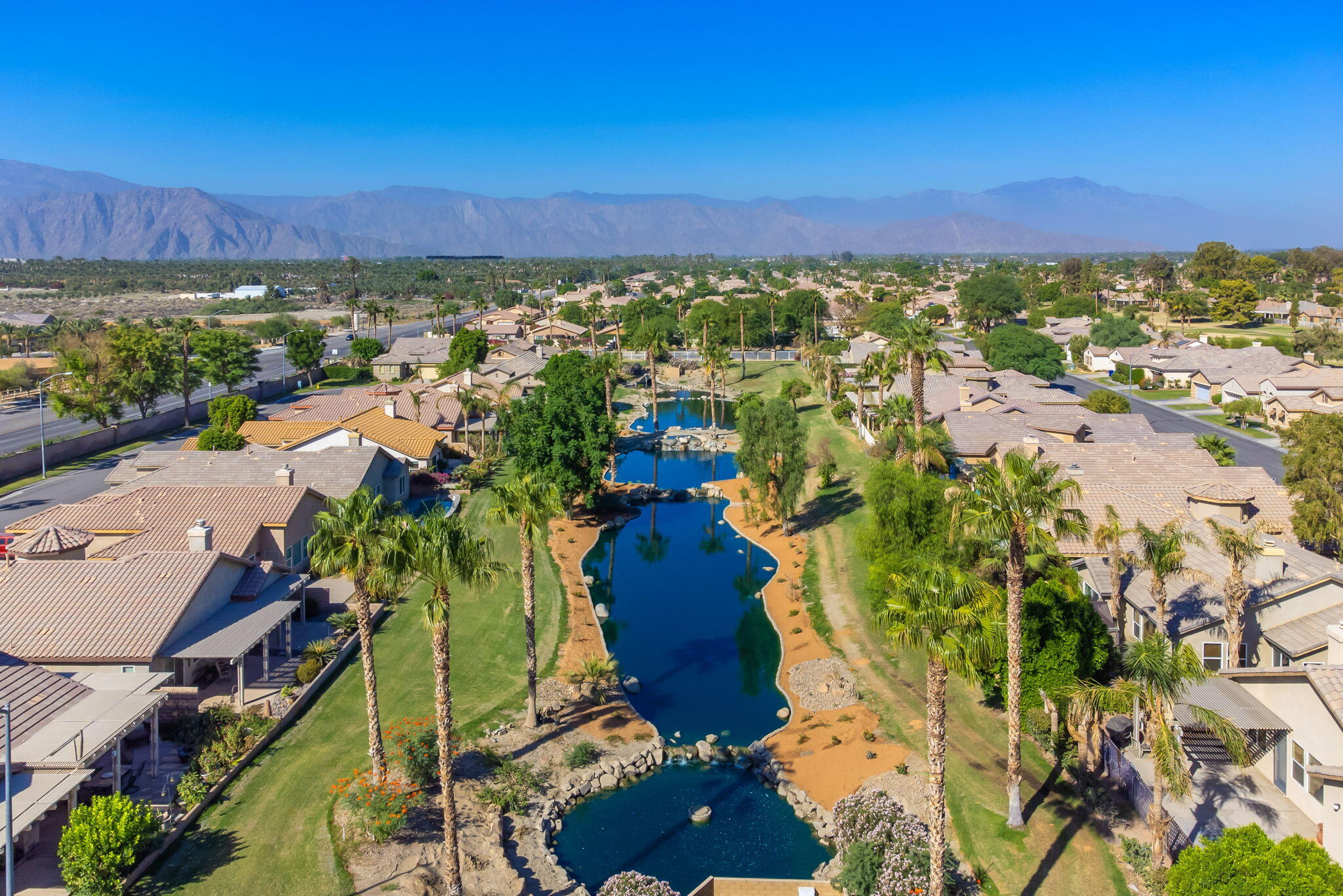This bright and clear photograph captures a sprawling suburban community nestled in what looks to be a desert or tropical environment. Palm trees dot the landscape, framing a series of ponds with strikingly blue water. The ponds are bordered by stones and surrounded by well-maintained, low-cut grass, indicative of meticulous upkeep, possibly by a homeowners' association. The homes in the community are uniformly built, suggesting they were constructed around the same time, adhering to specific design specifications aimed at weather resilience. This standardized, yet subtly varied architecture hints at a managed development, common in Californian or southwestern U.S. suburbs. Rugged, hazy blue mountains rise in the far distance, behind a vast flat plain that extends from the homes. The surrounding greenery stretches towards these mountains, adding depth to the serene backdrop. The scene is crisscrossed by several roads leading away from the development, with a prominent wall and wider highway visible to the left. The sky above is a stunning, unblemished blue, emphasizing the clarity and warmth of the day.